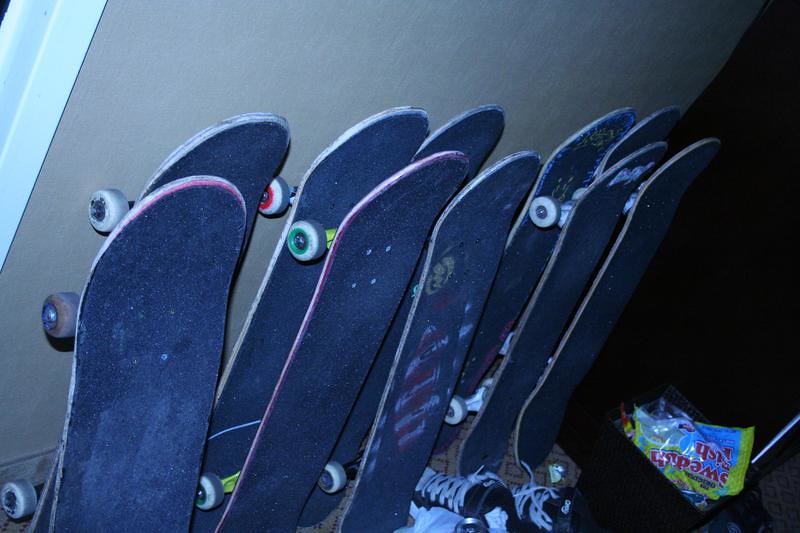This photo captures a dimly-lit room with a focal point on ten skateboards leaned against a smooth, solid gray wall with white crown molding on the left-hand side. The tops of the skateboards, covered in a rough black, sandpaper-like material, face the viewer, while their variably colored wheels, such as white and black with green and red centers, touch the wall. At the floor's edge, there’s a pair of large black tennis shoes with white laces positioned among the skateboards. In the bottom right corner stands a trash bin filled with rubbish, most notably a plastic Swedish Fish wrapper displaying green borders and some blue coloring. Behind the trash bin, a large black cabinet or appliance extends into the backdrop, adding to the room's details.